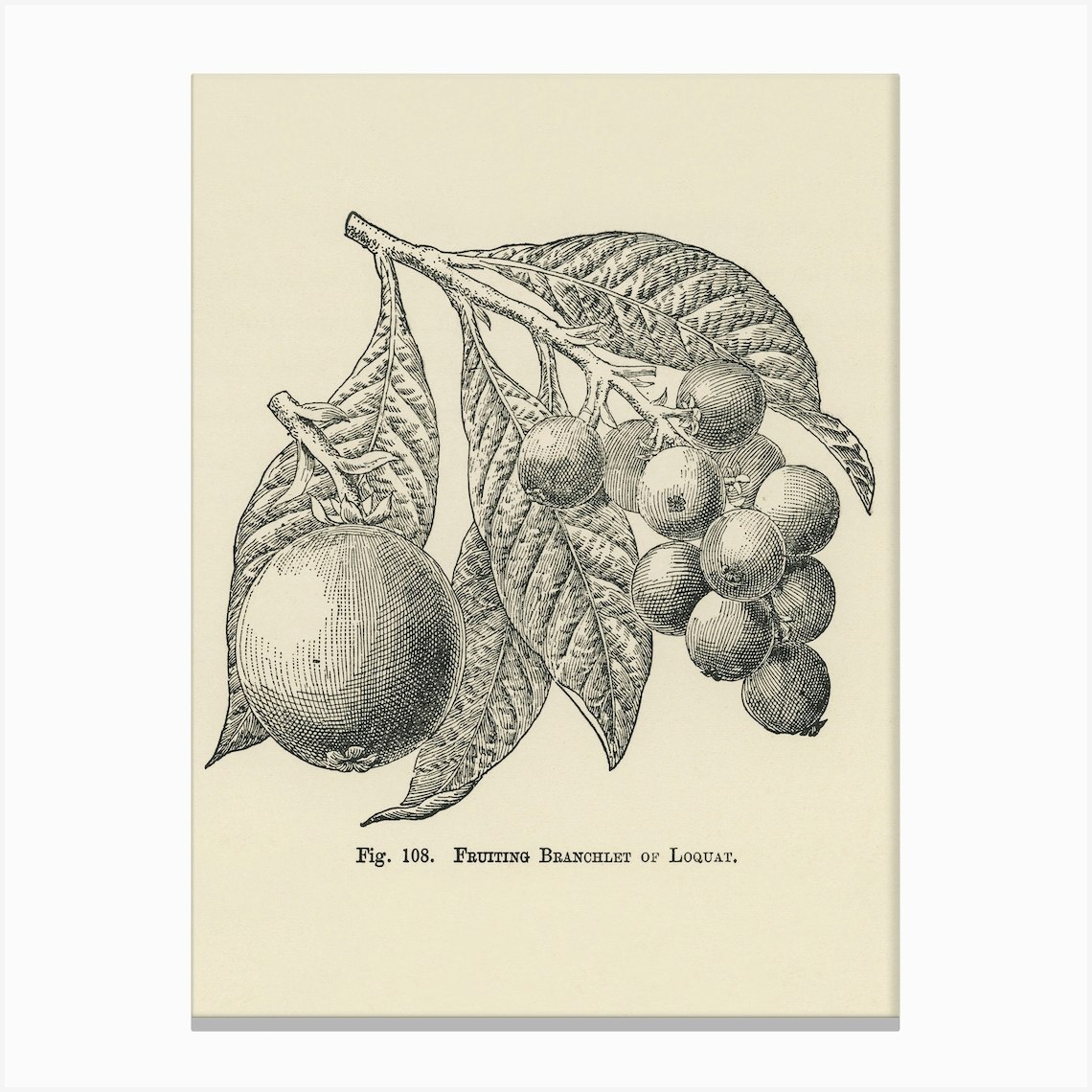This detailed, botanical illustration, reminiscent of an old textbook drawing, depicts a fruiting branchlet of a loquat with intricate cross-hatching. The black-and-white sketch, set against an off-white or beige background, shows a central stalk with four distinct, oval-shaped leaves. On the right end of the stalk, there's a cluster of smaller, spherical fruits that resemble grapes, complete with a small flower attached to one end of the bulbs. On the left, a larger round fruit is shown, which may be an enlarged view of the smaller fruits for detailed observation. The base of the image contains the text "Figure 108, Fruiting Branchlet of Loquat" in a faded serif typewriting font.